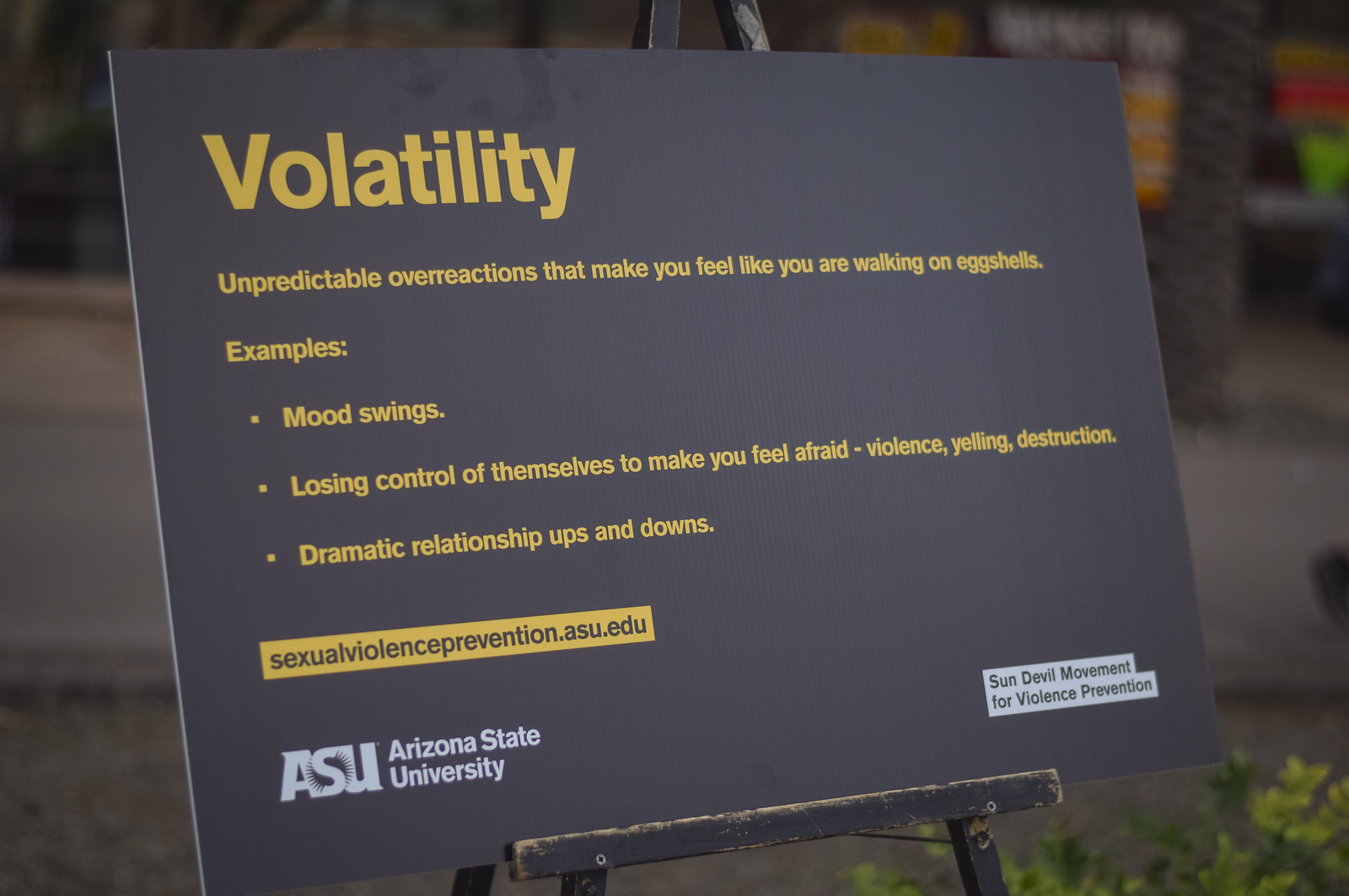The image shows a black poster displayed on a faded wooden easel set outside. The background is blurry with indistinct plants, trees, and possibly a sidewalk. The top of the poster reads "Volatility" in big, yellow letters. Below this, in smaller yellow letters, the text describes "unpredictable overreactions that make you feel like you're walking on eggshells," listing examples such as mood swings, losing control to instill fear, violence, yelling, destruction, and dramatic relationship ups and downs. Underneath, within a yellow rectangle, the text "sexualviolenceprevention.asu.edu" appears in black letters. The bottom of the poster features the ASU (Arizona State University) logo in white text alongside the name, and the phrase "Sun Devil Movement for Violence Prevention" in black text within white rectangles in the bottom right corner.